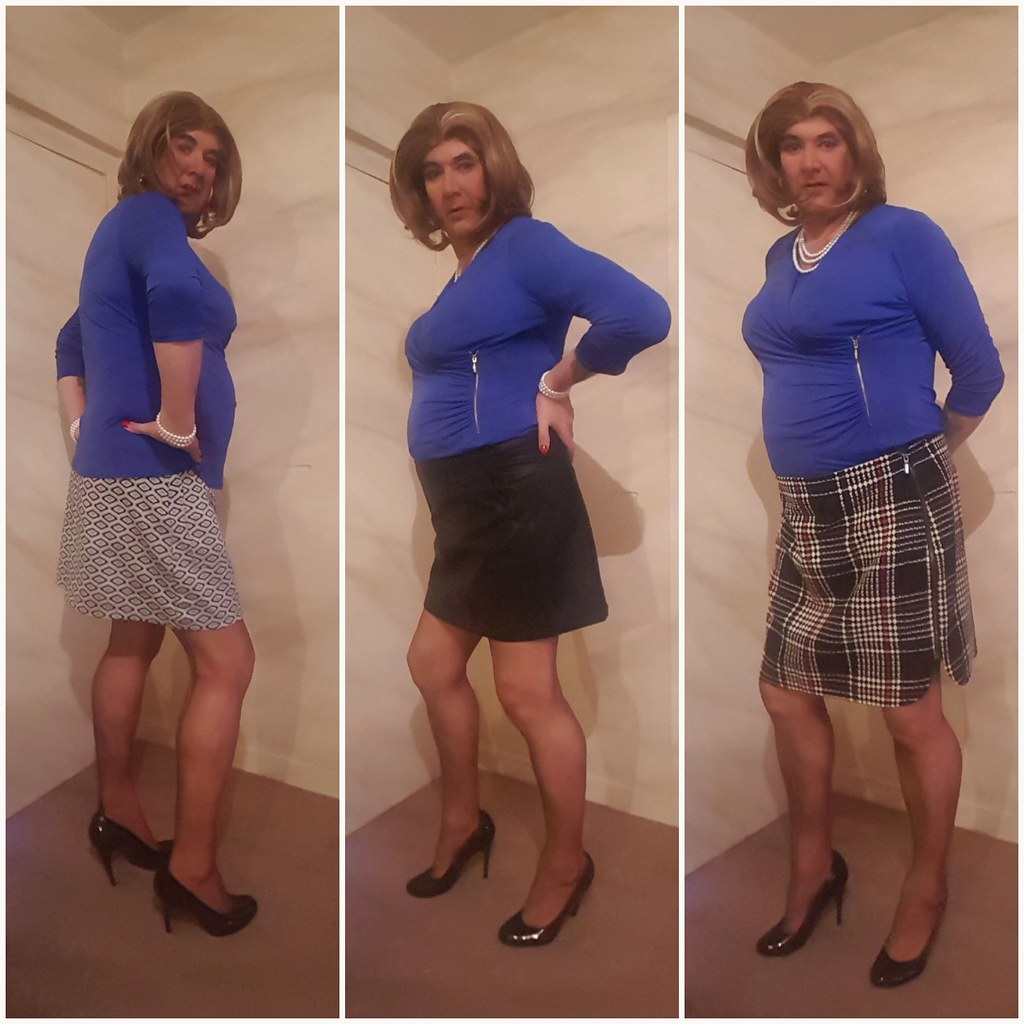A triptych photograph captures a trans woman posing in three distinct outfits within a white room featuring a brown floor. Each panel showcases her in the same outfit except for different skirts: a blue long-sleeved top with a zipper on the side, black pumps, and a shoulder-length strawberry blonde wig. In the left panel, she faces the camera while turning her body to the right, wearing a gray skirt adorned with a black diamond pattern. The central panel presents her in a profile view to the left, sporting a simple black skirt. The right panel depicts her in a plaid skirt with black, white, and hints of red, secured by a pin on her left hip. In all images, she accessorizes with a pearl necklace.